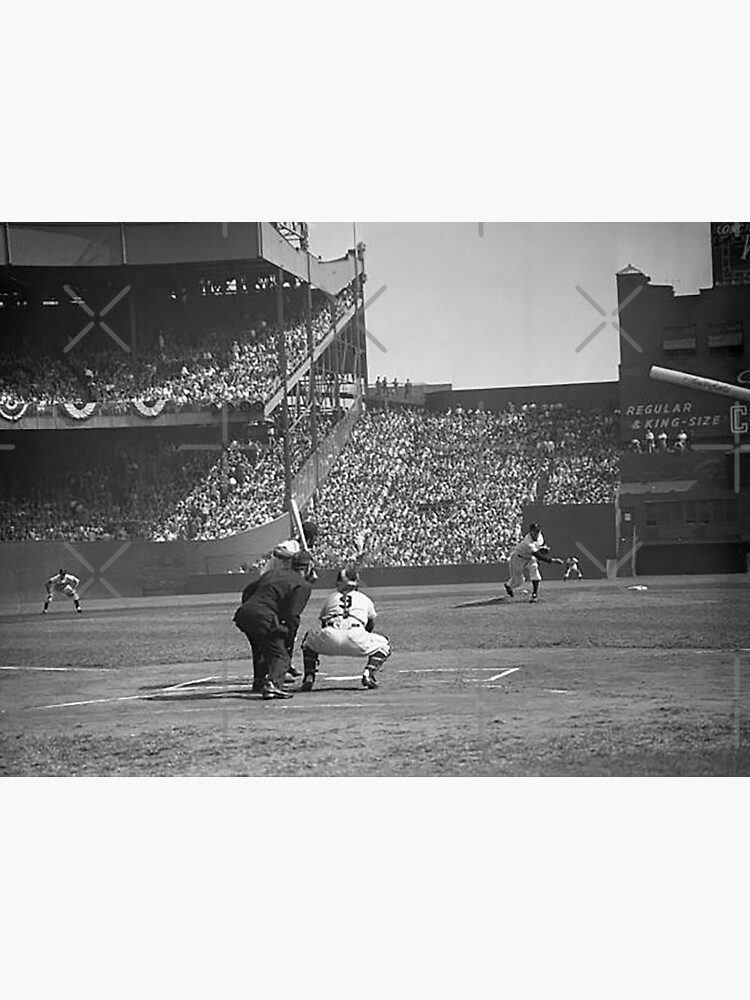In this black-and-white vintage photograph of a bustling baseball game, the rectangular image is bordered top and bottom with thick grey strips, each approximately one-fourth of the overall height. The photograph itself is in portrait orientation, with height twice that of its width. Captured from the perspective behind home plate, the image prominently features the catcher, crouching in an all-white uniform marked with the number nine. Behind him stands the umpire in an all-black suit and face mask, and in front, a right-handed batter poised to hit the ball. In the distance, the pitcher, wearing white with a dark cap, has just completed his pitch.

The background is dominated by an open-air stadium filled to capacity with spectators. On the left, a towering, double-decker bleacher section stretches skyward, while the center of the field is lined with a large, single-level grandstand. The right side features a scoreboard structure, emblazoned with advertisements reading "regular" and "king size." Above the upper deck of the bleachers is a roof providing shade, highlighting that the game takes place during daylight hours. The field also showcases the shortstop and center fielder, neatly completing the scene of this classic moment in baseball history. The image is overlaid with semi-transparent grey X watermarks at various intervals, subtly reminding viewers of its archival nature.